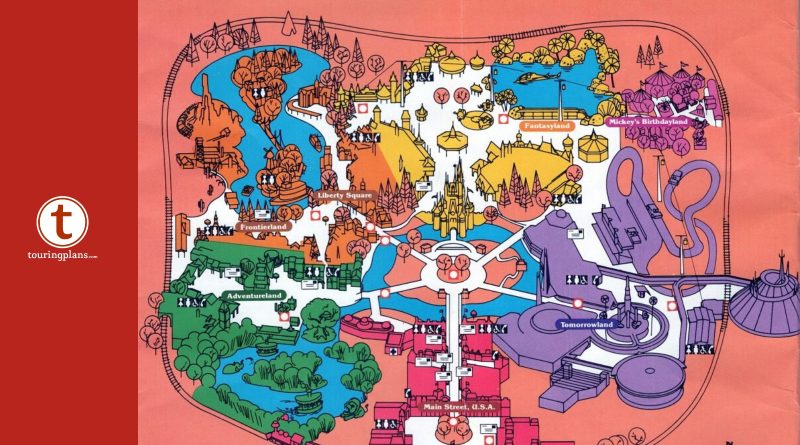The image is a rectangular digital map of a theme park, approximately six inches wide and three inches tall. On the left side, there's a red band with a white circle in the center, outlined in red, containing a lowercase red "T" and labeled "Touring Plans" underneath. The background of the map is a pinkish-orange shade. 

At the bottom center, there's an area labeled "Main Street USA," depicted with pink buildings and a white walkway extending to the center of the image. From the center, six spokes extend outward:

1. **Fantasyland** (Yellow, at the top center) features a castle.
2. **Mickey's Birthday Land** (Dark Pink, upper right corner).
3. **Tomorrowland** (Lavender Purple, mid-right).
4. **Adventureland** (Green, lower left).
5. **Frontierland** and **Liberty Square** (Brown, upper left).

Surrounding these areas are train tracks with a small train featuring Mickey ears in each section. The detailing includes various colors such as red, pinkish-orange, green, blue, purple, and yellow, giving it a vibrant, whimsical appearance reminiscent of a Disney World map.